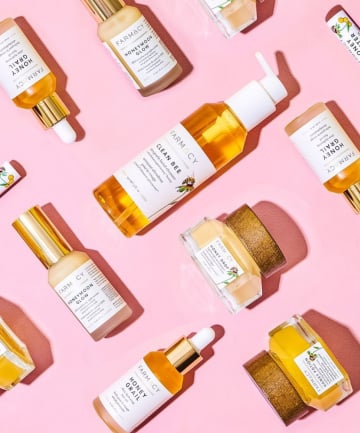The image is a rectangular photograph, taller than it is wide, featuring a meticulously arranged assortment of FarmCY beauty products against a bright, light to medium pink background. The setup appears to be intentionally designed for a professional marketing campaign, possibly for FarmCY's website or promotional emails. The products, which include items such as serums, droppers, pump bottles, screw-cap tubs, and chapsticks, are predominantly in a golden yellow or creamy golden yellow color, some with pale tan pink hues. The containers are strategically placed on their sides in a synchronized, grid-like pattern, with their white labels and branding, including names like "Honey Grail," "Honeymoon Glow," "Clean Bee," and "Honey Drop," all facing perfectly upward for optimal visibility. The screw-cap lids are notably brown, adding a contrasting detail to the setup. The overall composition is aesthetically pleasing, radiating a sense of organized beauty and elegance.